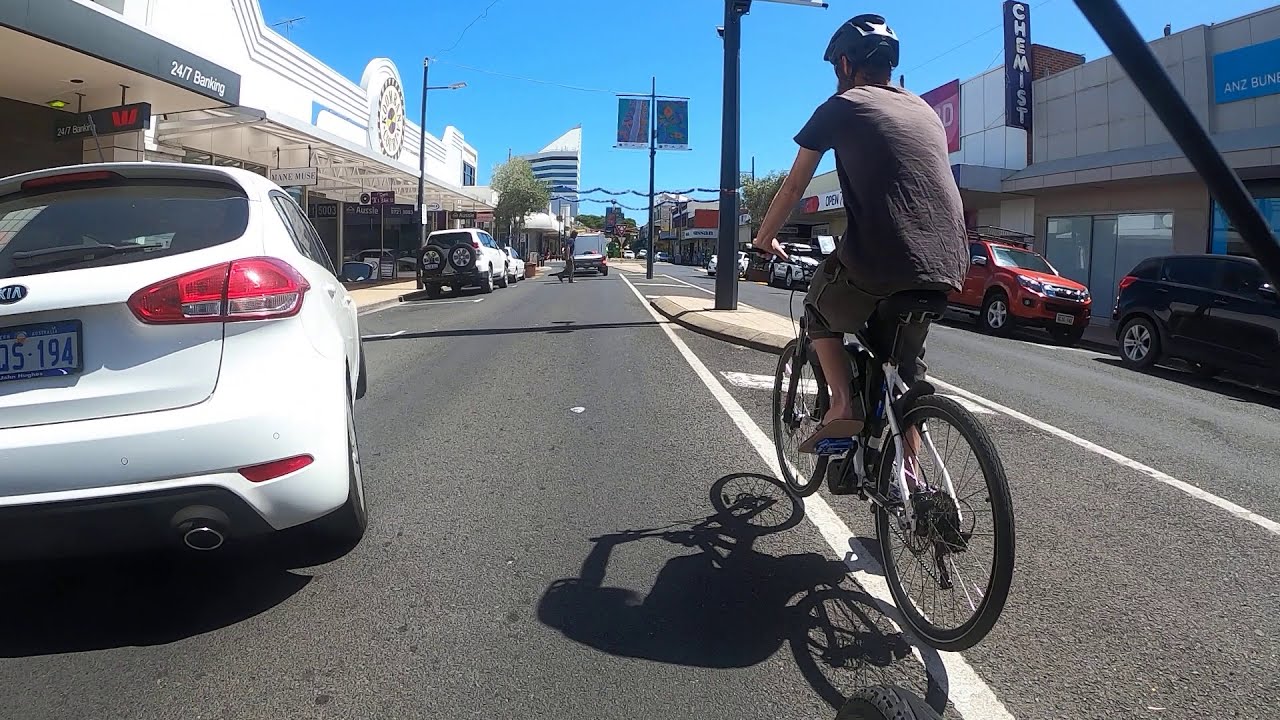In this urban street view, a man is prominently shown riding a white and black bicycle in the center of a two-lane road. He is dressed in a gray shirt, matching gray shorts, black helmet, and flip-flops. The lanes are divided by small concrete islands featuring dark gray pillars adorned with banners. To the left, a white car with a blue and white license plate bearing the characters S194 is pulling into a parking area, followed by a jeep with two spare tires mounted at the back. The setting appears to be an industrial downtown area or possibly a foreign country based on the left-side driving pattern. Behind the road, there are various commercial buildings including a 24-7 banking service with a red 'W', and further down, signs for "Aussie" and a chemist. The scene captures the essence of a bustling yet structured urban environment under a clear blue sky.